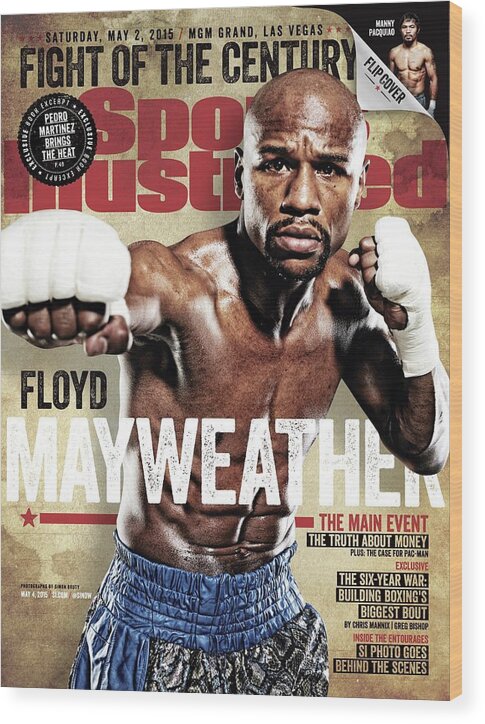This is the cover of the Sports Illustrated magazine dated Saturday, May 2, 2015, highlighting the "Fight of the Century" at the MGM Grand in Las Vegas between Floyd Mayweather and Manny Pacquiao. The cover prominently features a shirtless Floyd Mayweather, who is depicted punching his right arm towards the camera, with his gloves wrapped and his intense gaze fixed forward. He is wearing blue shorts with a black and silver-white trim. The headline reads "Floyd Mayweather" across his abdomen area, and additional cover text includes articles such as "The Main Event," "The Truth About Money," "Exclusive: The Six Year War, Building Boxing's Biggest Bout," and "SI Photo Goes Behind the Scenes." The right side of the cover is designed with a flip cover effect, revealing half of Mayweather's body.